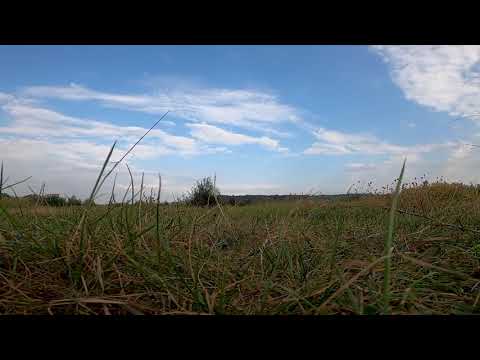The photograph features a close-up ground view of a grass field, dominated by strands of green and brown grass, some lying sideways. The camera appears to be placed at grass level, capturing the field from a unique perspective. On the left side and further back, the horizon meets a line of trees, with a prominent bush or a larger tree slightly to the left-center of the image. The right side of the horizon subtly rises, suggesting a small hill. The sky occupies the top half of the image and is predominantly blue with wispy cirrus clouds and possibly larger, distant clouds. The clouds extend across the sky, creating wave-like and snake-like formations. The photograph is framed with a black border on the top and bottom, each taking up about ten percent of the image's height. Despite its grainy, low-quality appearance, one might notice a hint of flowers on the right side, partially obscured by the grass. The focus is undeniably on the natural elements of the field and the sky.